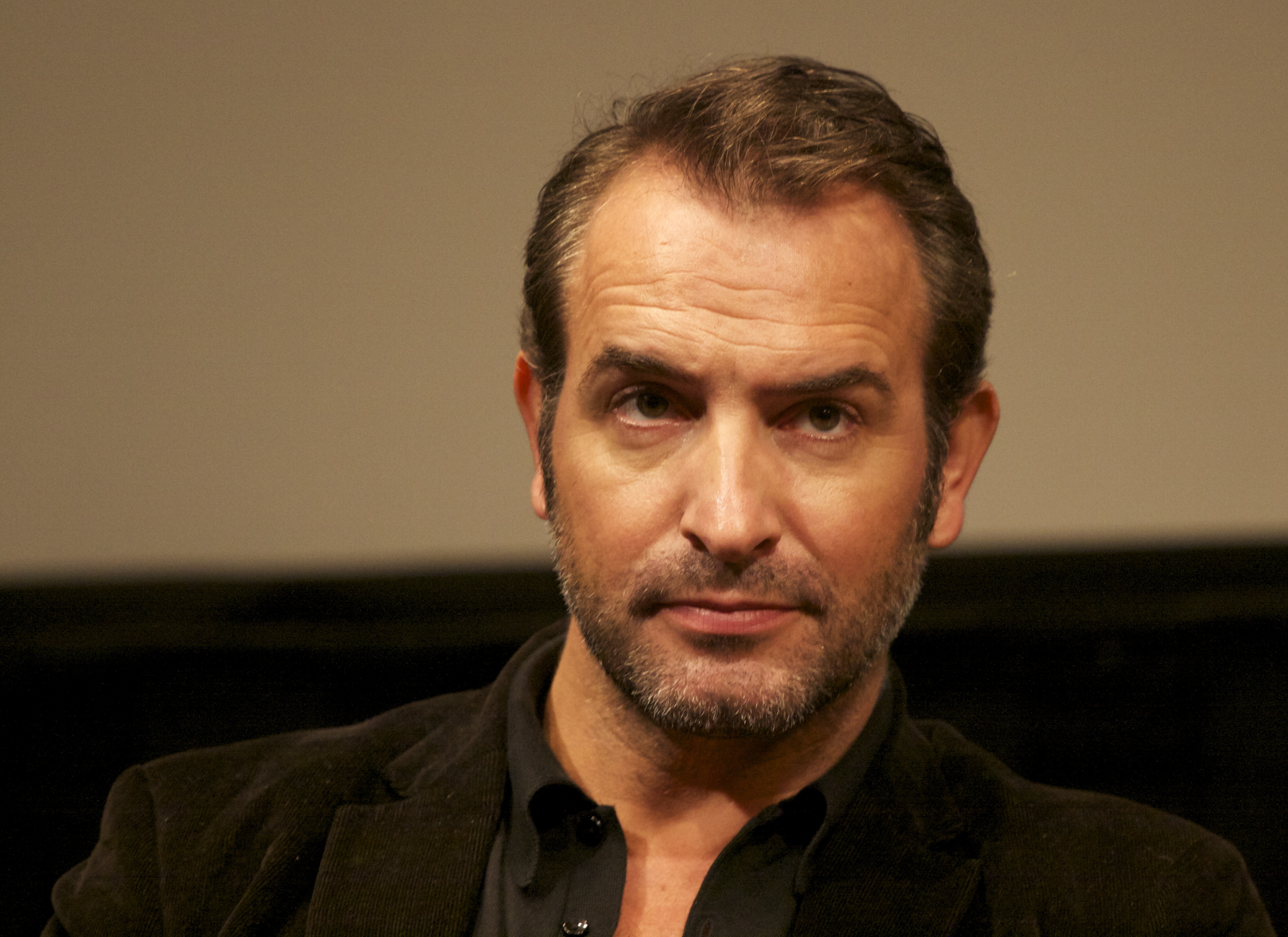This image prominently features a middle-aged Caucasian man, likely in his late 40s to early 50s, with a serious expression. The photograph is zoomed in to show only his head and shoulders. He has wispy, blondish-brown hair with some gray around the temples and a receding hairline. His facial hair consists of a white stubble that's part of a salt-and-pepper beard and mustache. The man is looking slightly to the left, his head tilted slightly, making his head appear closer to the right side of the image while his shoulders are centered. He has dark-colored eyes and a few wrinkles on his forehead, suggesting a more mature age. He is dressed in a dark button-down collared shirt under a dark brown or gray jacket. The background is a solid beige or light coffee brown color, creating a simple, unobtrusive backdrop that ensures he remains the focal point of the image.